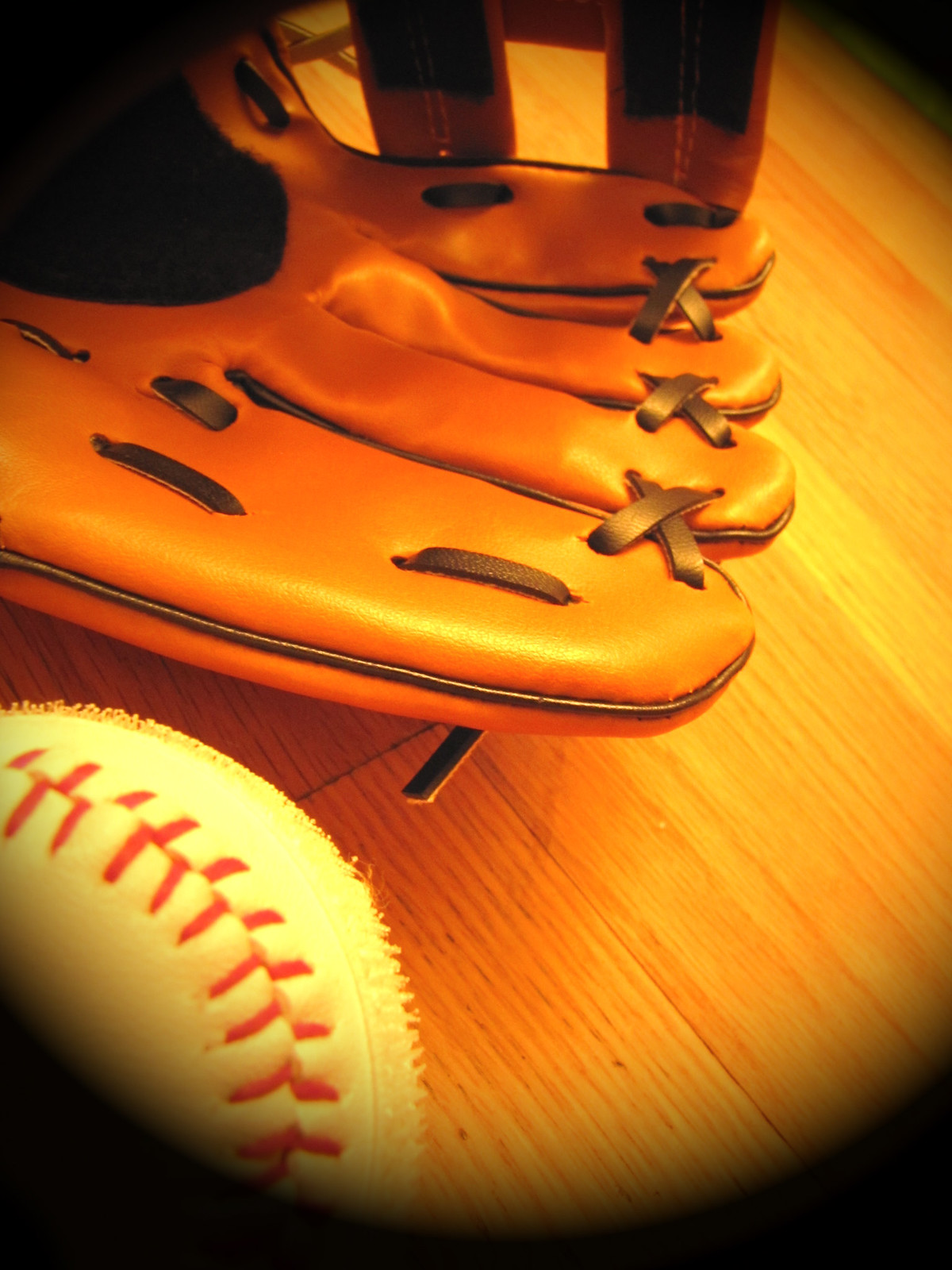The image captures a nostalgic, almost sepia-toned scene with a golden light cast over what appears to be a new leather baseball mitt and a white baseball with red stitching. The background features a red oak or similar wooden floor, bathed in light and subtly faded around the edges, as if viewed through a peephole or portal, adding a sense of focus and intimacy to the shot. The baseball mitt, positioned centrally and slightly to the left, is a light brown color with dark brown stitches, possibly vinyl, and appears very clean and unused. The mitt is open with the palm facing up, prominently displaying the finger slots designed to create a cohesive and sturdy catching area. Below the mitt, towards the lower left, lies the baseball. While the mitt dominates the scene, the baseball, though small in comparison, stands out due to its striking whiteness and red stitching, contributing to the clean and pristine aesthetic shared by both objects.